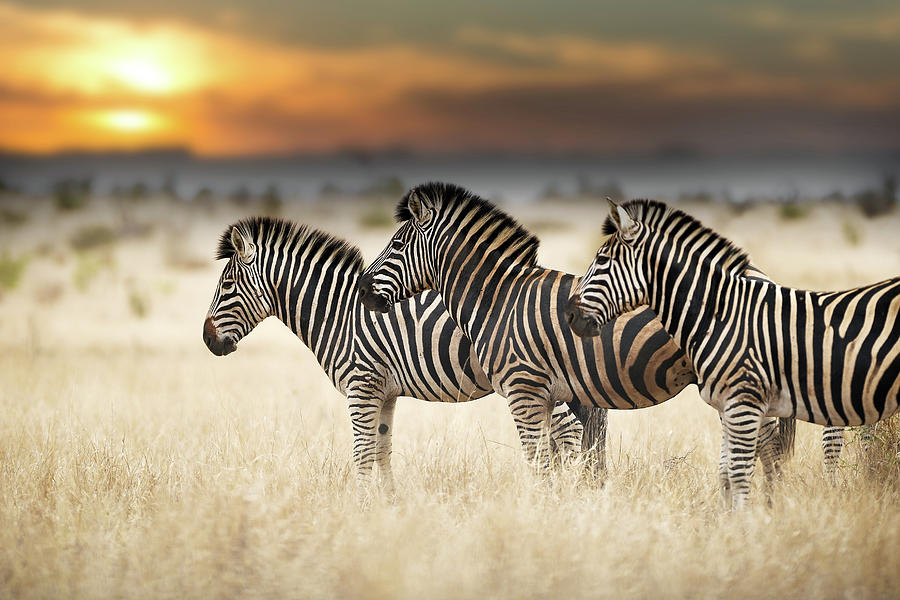In this horizontal landscape photograph, three zebras stand side by side in a large expanse of tall, tan, wheat-like grass that reaches up past their knee joints. Captured during the day with the sun peeking through a break in the clouds in the upper left-hand corner, the image showcases a serene and expansive outdoor scene. The dry grass covers much of the ground, and the horizon features low hills in the distance. The zebras, all facing left and aligned in a line, display their iconic black and white stripes clearly from a side view, with one eye, one ear, and their nose visible. The sky above is filled with gray clouds with a hint of yellow where the sunlight breaks through, enhancing the tranquil sunset atmosphere.